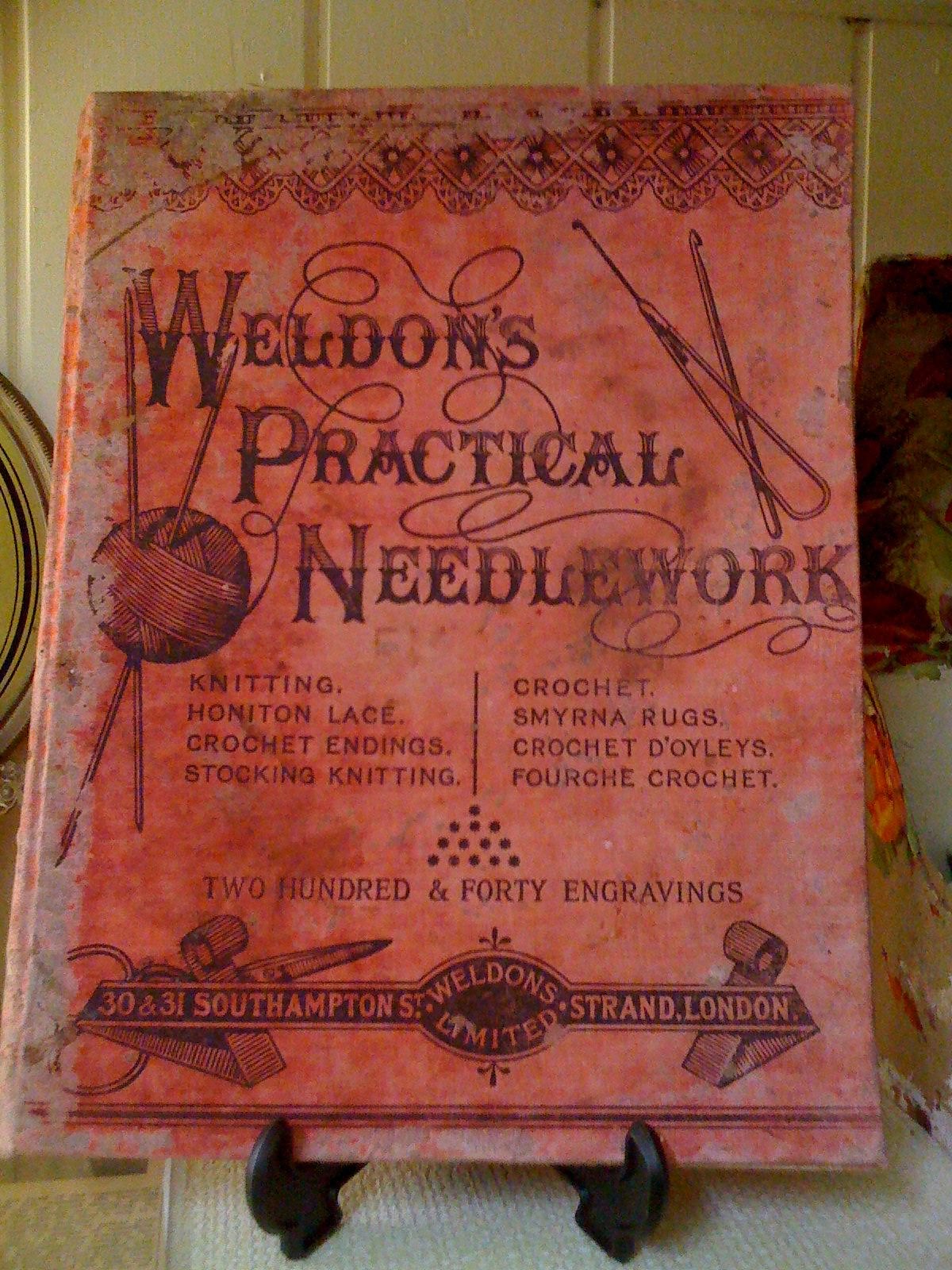In the center of the vertically-oriented photograph, an aged and heavily worn hardback book is displayed on a black hammer-shaped stand. The book, which once had a red or pink cover, is now frayed and faded, revealing underlying brown and grey tones. The title and details on the cover are printed in black text, which includes "Walden's Practical Needlework" prominently at the top, followed by "Knitting, Honiton Lace, Crochet Endings, Stocking Knitting, Crochet, Smyrna Rugs, Crochet Doilies, Fourchette Crochet." A decorative lace pattern adorns the top, complemented by an illustration of a ball of yarn with two knitting needles emerging from it, with a single thread weaving throughout the title. Below, the book mentions "240 Engravings," and across the bottom, it lists the address "30 and 31 Southampton Street, Strand, London" with the publisher "Weldon's Limited." In the background, light yellow patterned wall panels and a piece of furniture such as a sofa or chair are partially visible, completing the scene.